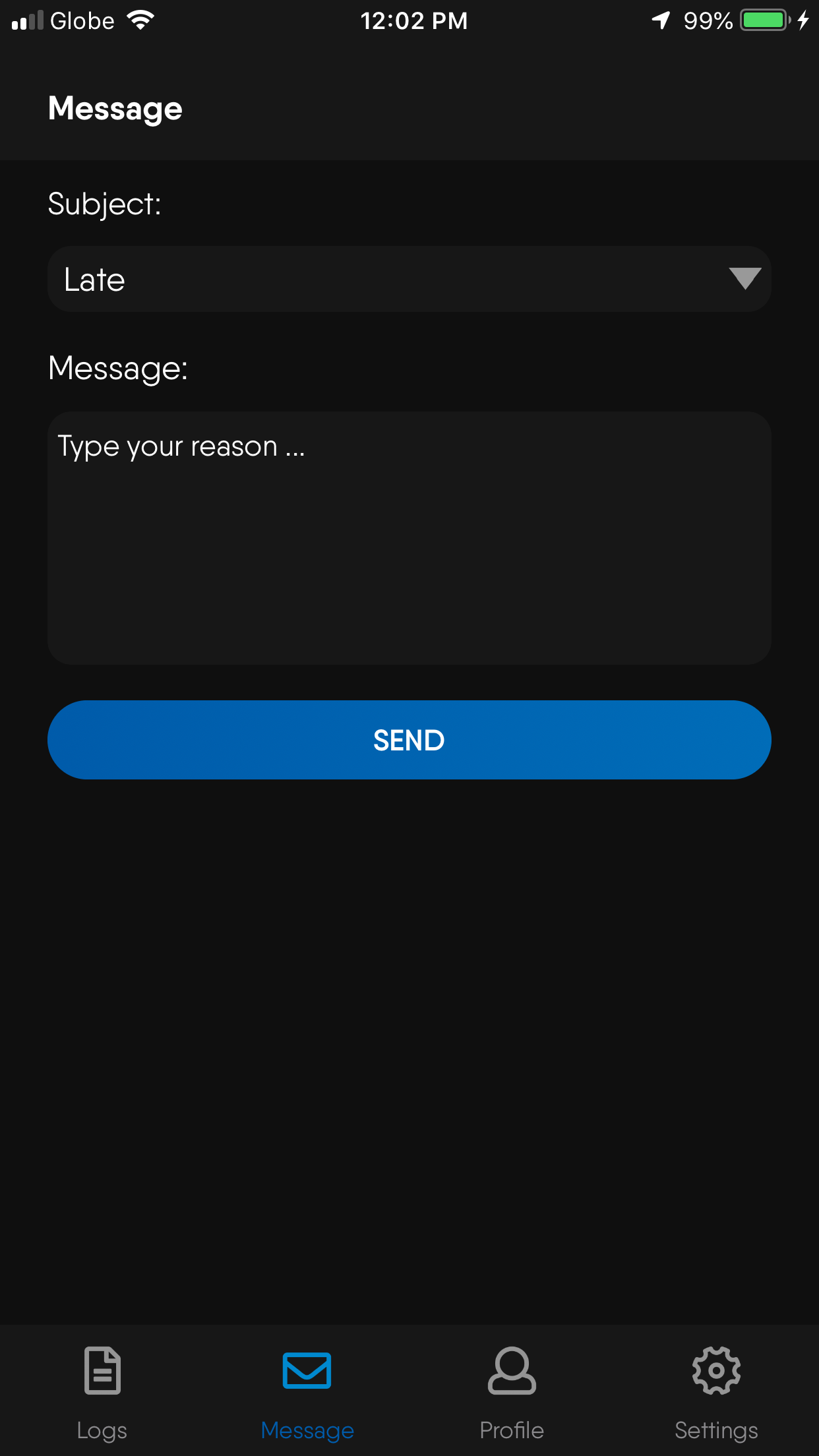The image depicts a smartphone interface with a black background. In the upper left corner, there are four signal bars with the first two bars filled in white while the other two bars are blank. To the right of the signal bars, the word "Globe" is displayed, followed by a white Wi-Fi signal icon. Centrally, the time is shown as 12:02 p.m. On the far right, a green battery icon indicates a 99% charge.

In the upper section of the screen in white text, the label "Message" is prominently displayed. Below this, there is the word "Subject:" followed by a dropdown menu option labeled "Late." Farther down, a heading reads "Message:" accompanied by a light gray text box which contains the placeholder text, "Type your reason..." in white. Beneath the text box, a blue "Send" button stretches the full width of the text box.

The lower portion of the screen is dominated by a large black space. At the very bottom, there are four icons: a piece of paper with two lines labeled "Logs," a blue envelope icon labeled "Messages," a person icon labeled "Profile," and a gear icon labeled "Settings."

This detailed description provides a clear visual understanding of the smartphone interface design and its various elements.